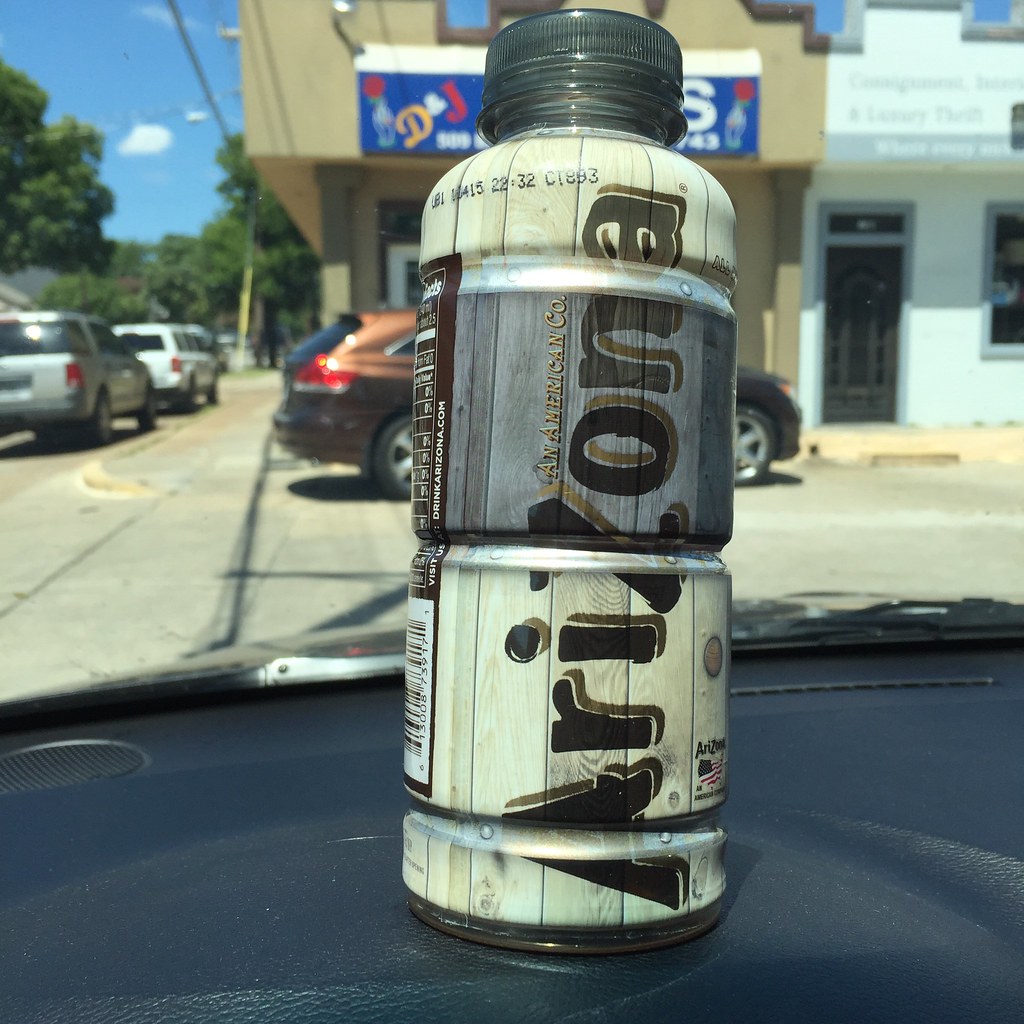Close-up of an Arizona Beverage Bottle on a Car Dashboard

This detailed close-up photograph captures a bottle of an Arizona beverage, presumably Arizona Tea, prominently displayed on the dashboard of a car. The bottle features the recognizable branding of Arizona, with the logo written vertically in black letters on a background that resembles painted wood. However, the specific type of tea or beverage is not legible in the image. The bottle is capped and positioned in a way that suggests the photo was taken by someone seated inside the car, looking outward through the windshield.

In the background, the windshield wipers are visible, indicating the car is stationary. The scene outside reveals a sunny day with a partially blue sky, accompanied by lush green trees. Directly in front of the car is a brown, copper-colored vehicle. Further down the street, there is a gray pickup truck and a white vehicle, with a building situated adjacent to the brown car. The image exudes a casual, everyday moment, enhanced by the presence of other cars and the sunny weather.